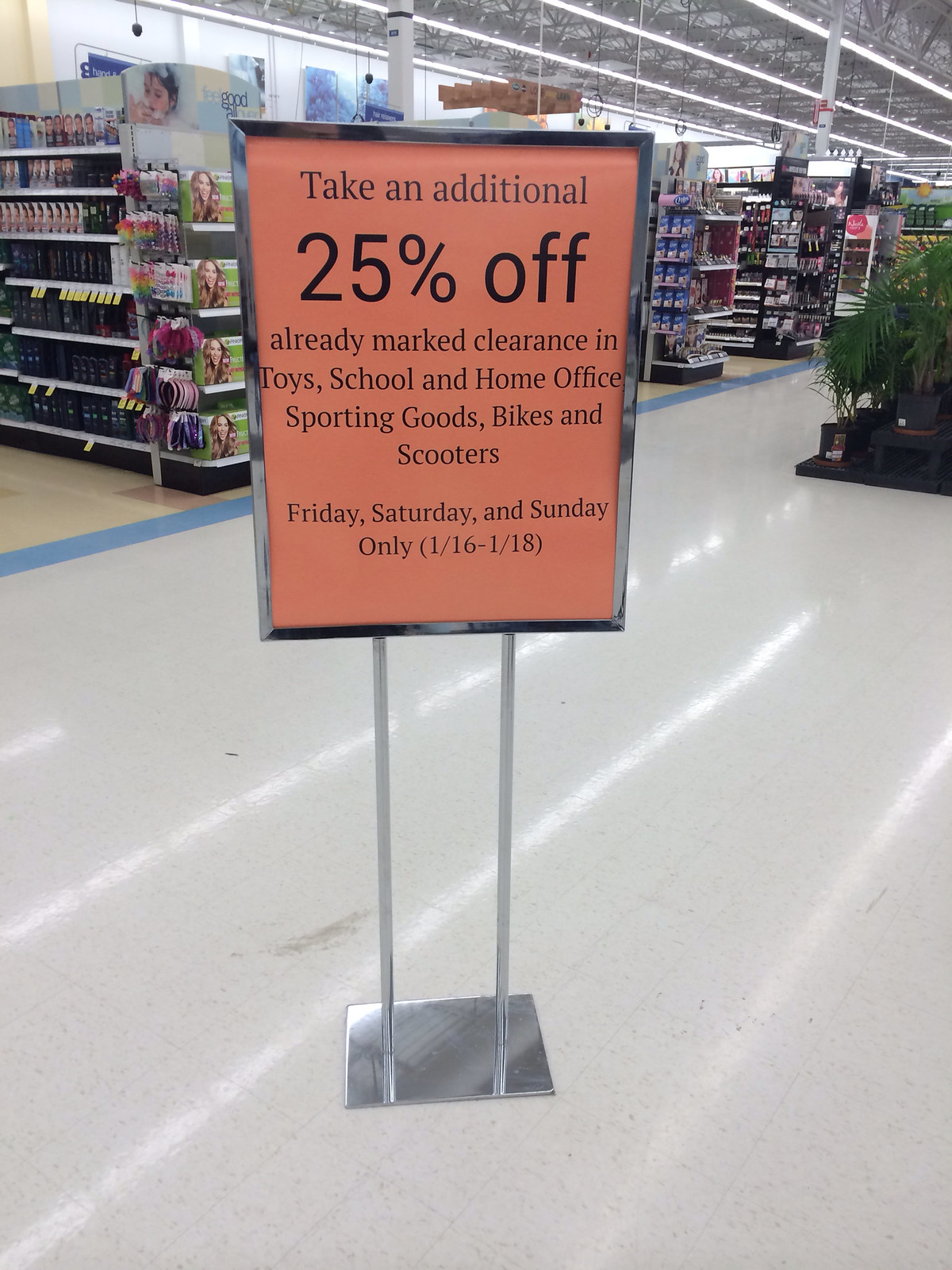The image shows a well-lit interior space with white tiling that reflects the overhead lights, creating a bright and clean atmosphere. In the background, there's a section of brown wooden panels, adding a touch of warmth to the decor. Various products are on display, including what seems to be hair coloring items and several skincare products organized neatly on shelves. Additionally, some potted plants with green leaves bring a bit of nature into the scene.

Prominently displayed at the front is a sign on an orange background with a silver metal border. The sign reads: "Take an additional 24% off already marked clearance on toys, school and home office supplies, sporting goods, bikes, and scooters. Friday through Saturday only (1/16 - 1/18)." Below this sign, there are two metallic legs supporting another silver structure at the bottom.

The overall setting appears to be a retail store, possibly a section dedicated to beauty and wellness products, with promotional discounts highlighted for certain categories.